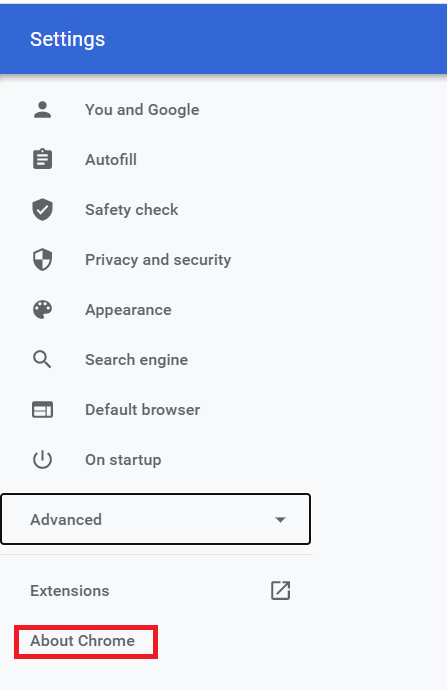Screenshot of Google Chrome Settings Page:

The image displays a screenshot of the Google Chrome settings page. At the top, a blue header contains the word "Settings" in white text, accompanied by a pronounced drop shadow for added depth. Below the header, several icons represent various settings categories, each accompanied by descriptive text:

- A person icon followed by "You and Google."
- A clipboard icon with "Autofill."
- A check mark symbolizing "Safety check."
- A shield denoting "Privacy and security."
- A palette representing "Appearance."
- A magnifying glass illustrating "Search engine settings."
- An icon resembling a browser window signifying "Default browser."
- A power icon indicating "On startup."

Further down the page, a drop-down menu labeled "Advanced" is selected but not expanded. Below this, "Extensions" is listed alongside a pop-out arrow within a square, and "About Chrome" is highlighted with a thick, sharp-cornered red outline. 

The entire page rests on a white background, with most elements displayed in various shades of black and gray, except for the blue header, which stands out as the only colored item. The icons are simple grayscale graphics that are clear enough to convey their intended function.

The red outline around "About Chrome" was added post-capture for emphasis. The design is minimalistic, relying on grayscale icons and sans-serif text to maintain clarity and simplicity.